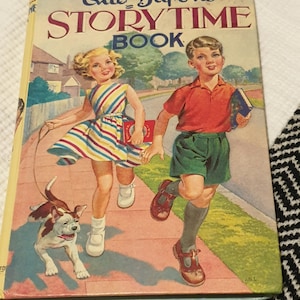This is a close-up photograph of the cover of an older, vintage-looking children's book titled "Storytime Book." The title is prominently displayed at the top. The cover illustration features a little boy and a little girl skipping down a terracotta-colored, clay sidewalk, possibly in their neighborhood. The boy is dressed in green shorts, knee-high socks, brown shoes, and a red shirt, and he is clutching a book under his arm. The girl, dressed in a white dress adorned with colorful stripes of red, blue, and yellow, wears white shoes and socks. She is holding a red book in one hand and a leash in the other, which is attached to a small white dog with brown spots that appears to be running alongside them. The illustration has a cartoonized style that adds a charming, whimsical feel to the vintage cover.